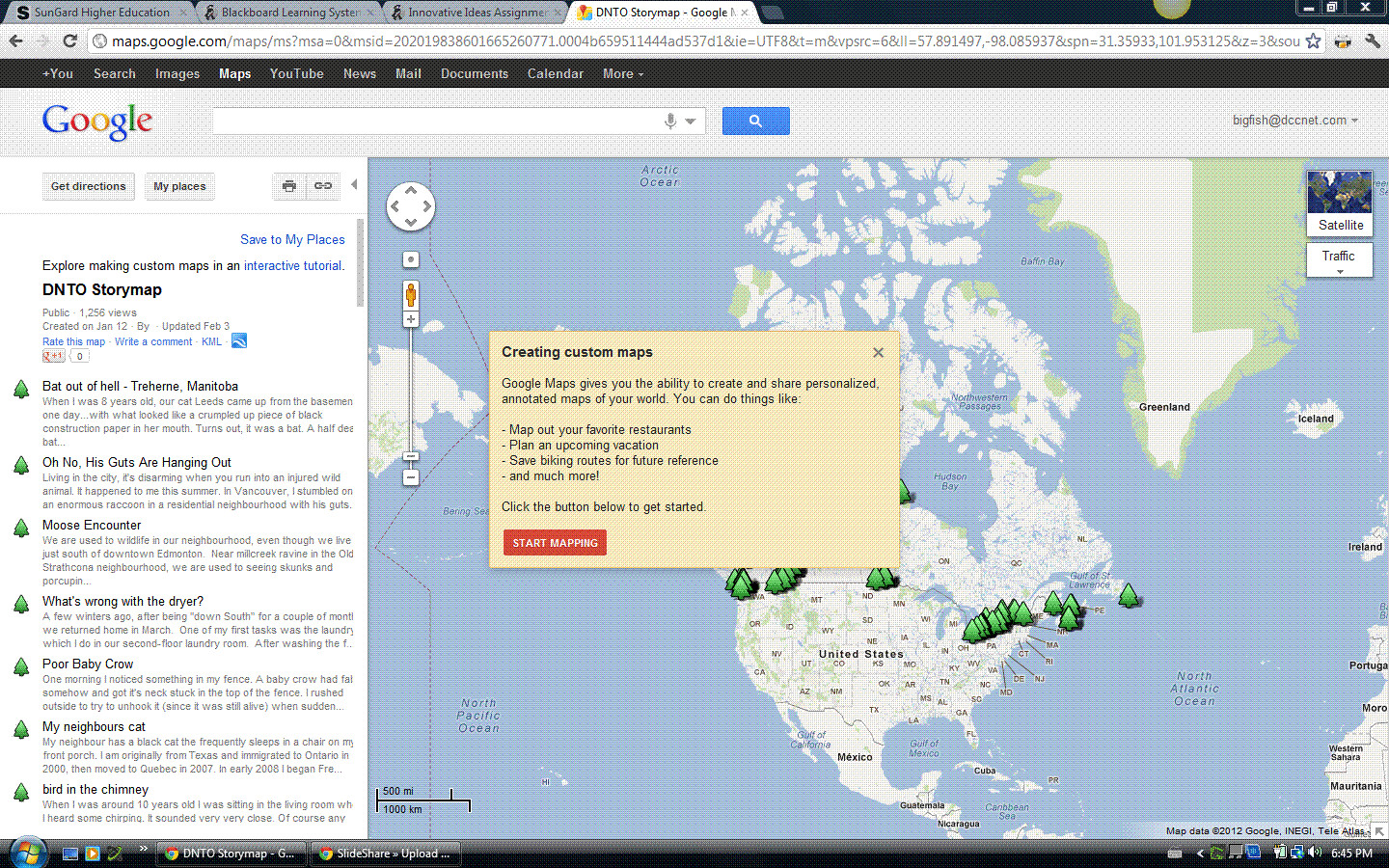A screenshot of a computer displaying a zoomed-out view of Google Maps, revealing the entirety of the United States and Canada. However, a large placard obscures most of Canada. The placard reads, "Creating Custom Maps: Google Maps gives you the ability to create and share personalized annotated maps of your world." It then offers suggestions on how users can utilize these features. 

On the left-hand side of the screen, there is a menu titled "DNTO Story Map." The map features numerous tree symbols, resembling Christmas trees, predominantly scattered around the US-Canadian border. These icons correlate with the entries listed in the left-hand menu, suggesting an interactive story map titled DNTO.

The computer appears to be running a Windows operating system, confirmed by the visible Start menu in the bottom left corner of the screen.